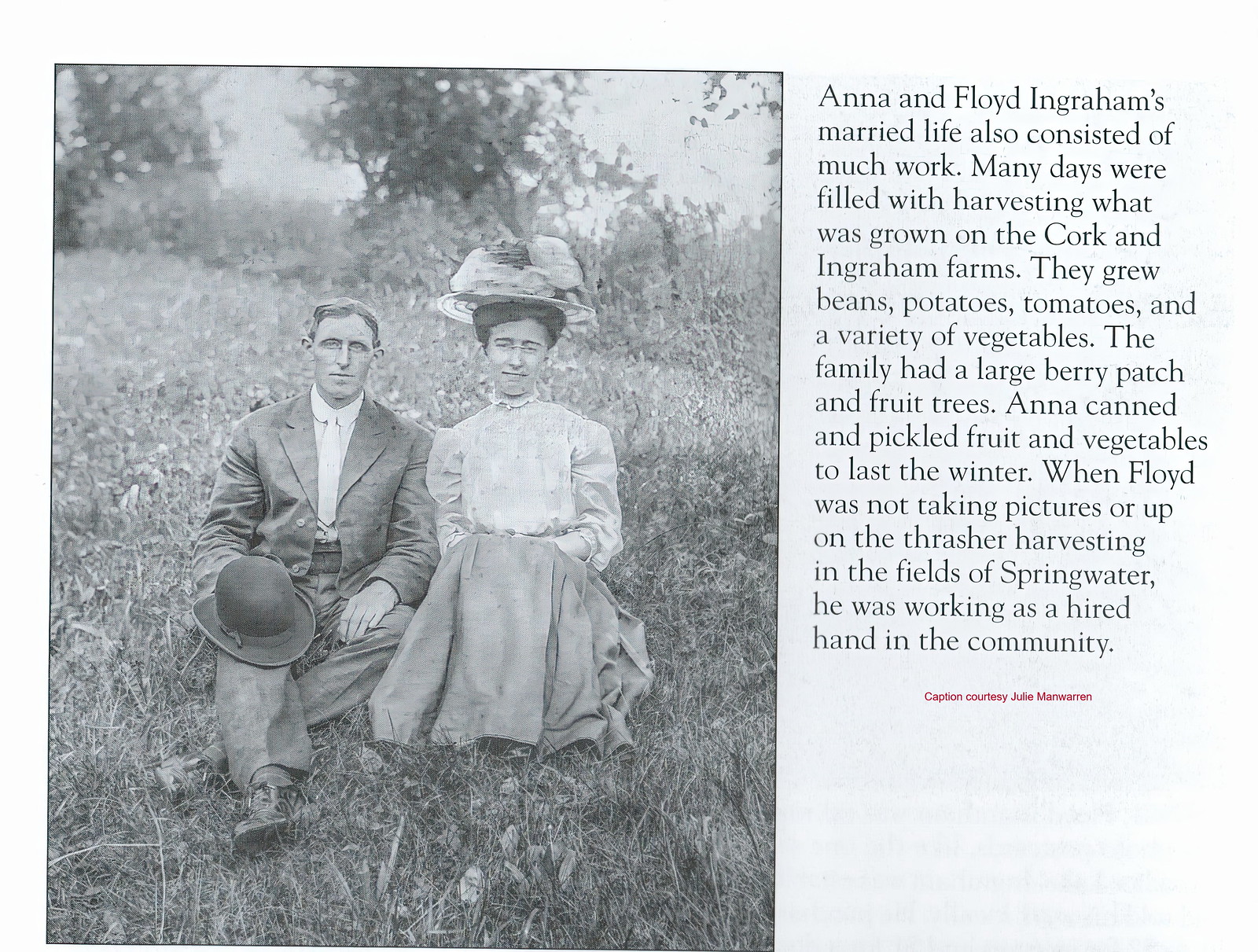The black-and-white image, likely an insert from a book, shows a young man and woman seated in a grassy field with trees in the background. Both are dressed in turn-of-the-century clothing; the man wears a suit and has a bowler hat on his right knee, while the woman dons a white blouse with a full skirt and a fancy, flower-adorned hat. Text to the right reads, "Anna and Floyd Ingram's married life also consisted of much work. Many days were filled with harvesting what was grown on the Cork and Ingram farms. They grew beans, potatoes, tomatoes, and a variety of vegetables. The family had a large berry patch and fruit trees. Anna canned and pickled fruit and vegetables to last the winter. When Floyd was not taking pictures or working on the thresher harvesting in the fields of spring water, he was working as a hired hand in the community. Captioned courtesy of Julie Manwarren." The image captures a historical snapshot of their hardworking rural life and commitment to self-sufficiency.